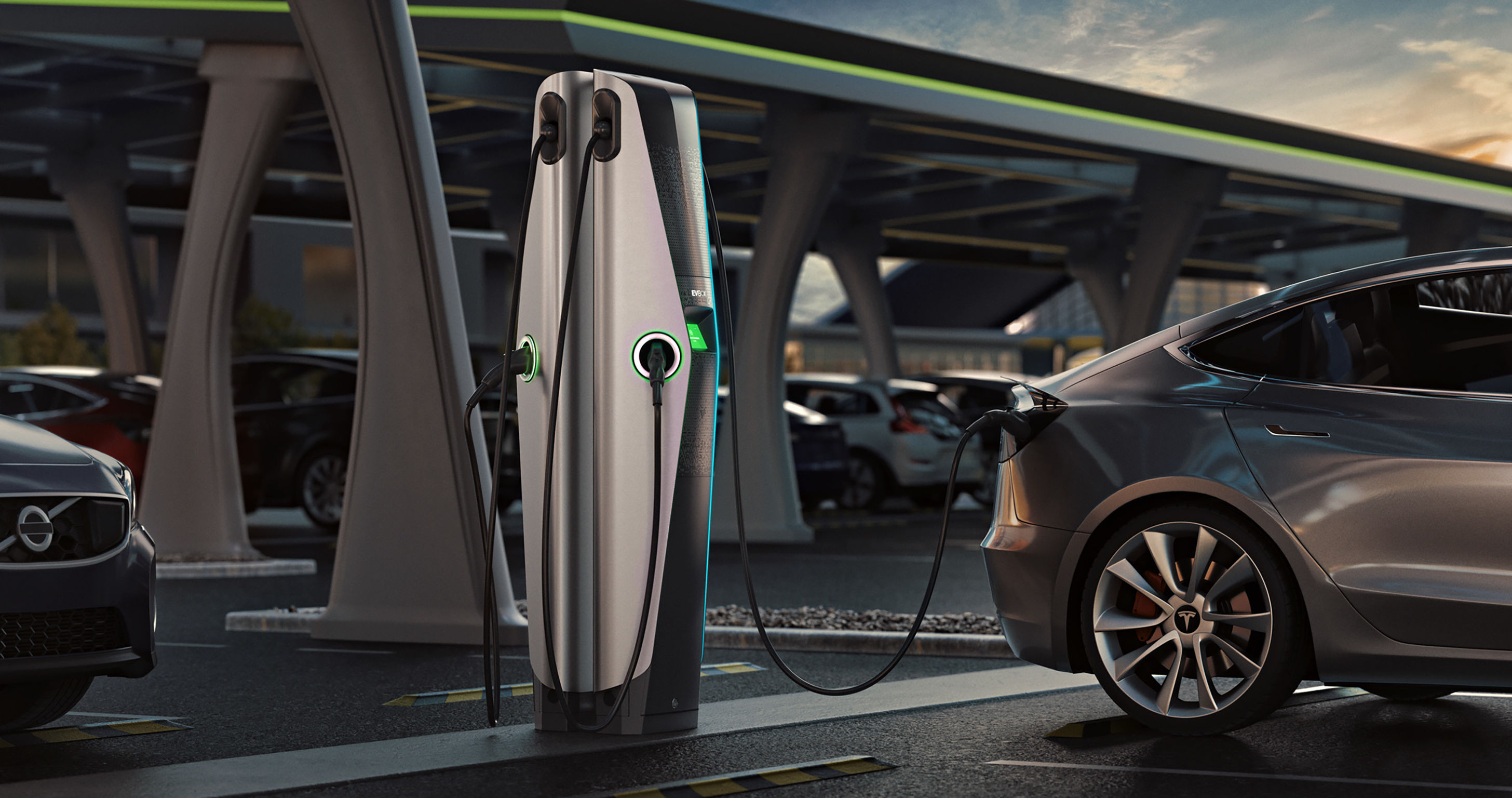The image captures a sleek and shiny, relatively new gray Tesla electric vehicle being charged at a futuristic, tall, and silver charging station equipped with distinctive circular cutouts housing black charging cords. The car's black windows, large silver rims, and the prominent Tesla logo on the back wheel rim are clearly visible. Positioned outdoors, the scene is set under a light blue sky with wispy white clouds, indicative of late evening light. The charging station, centrally located, stands beneath a slanted rooftop with gray pillars, part of an overhead solar array designed to provide shelter and harness solar energy for charging. Other vehicles are parked nearby, hinting at a well-equipped and modern parking facility designed specifically for electric vehicles.